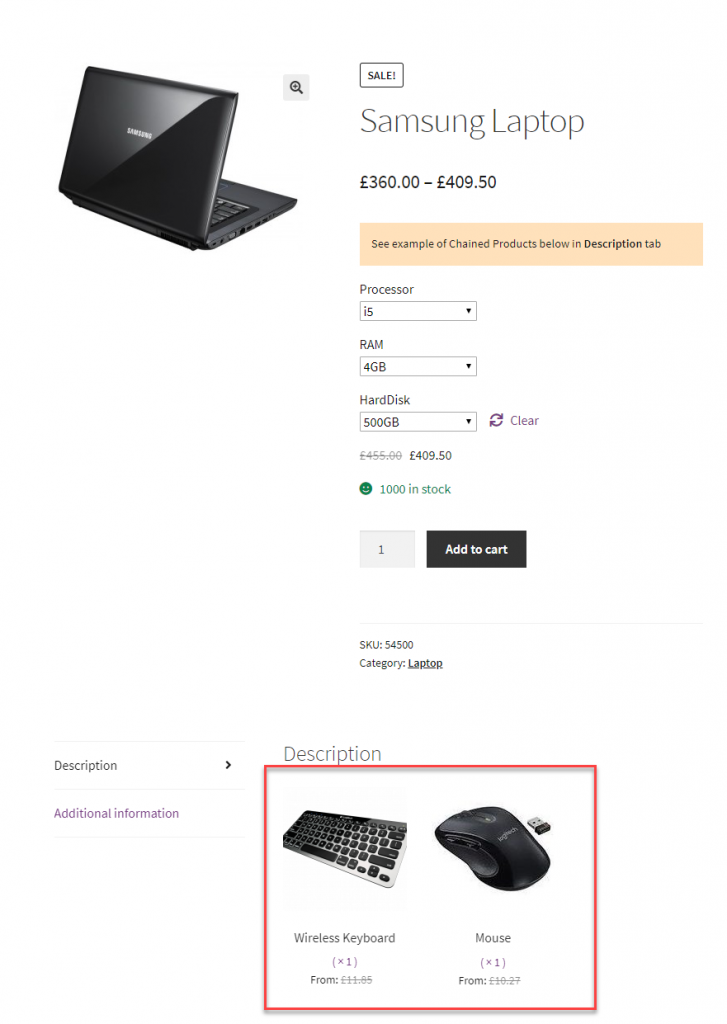Here is a cleaned-up and detailed descriptive caption based on the provided information:

--------------------------------

The web page features a prominent sale banner at the top, advertising a Samsung laptop. To the left, there's an image of a sleek black Samsung laptop. Below the "Samsung Laptop" heading, the price range is displayed, showing €360 to €409.50. The text advises visitors to see examples of chain products in the description tab.

The specifications section follows, listing the key features of the laptop:
- Processor: Intel Core i5
- RAM: 4GB
- Hard Disk: 500GB

A note indicates a price reduction, with an original price of €455 struck through and the sale price of €409.50 displayed prominently. The stock information states that 1000 units are available. Buyers can enter a quantity in a box (default set to 1) and click an "Add to Cart" button. The SKU for the product is 54500, and it falls under the category of laptops.

Beneath this section, there's a red-highlighted box featuring an image of a wireless keyboard and mouse. The caption for this image mentions that it's a "Wireless Keyboard and Mouse" set. There's a description tab on the left with an arrow pointing to additional information on the right. Underneath the wireless keyboard and mouse section, it further specifies "1x" with a corresponding price.